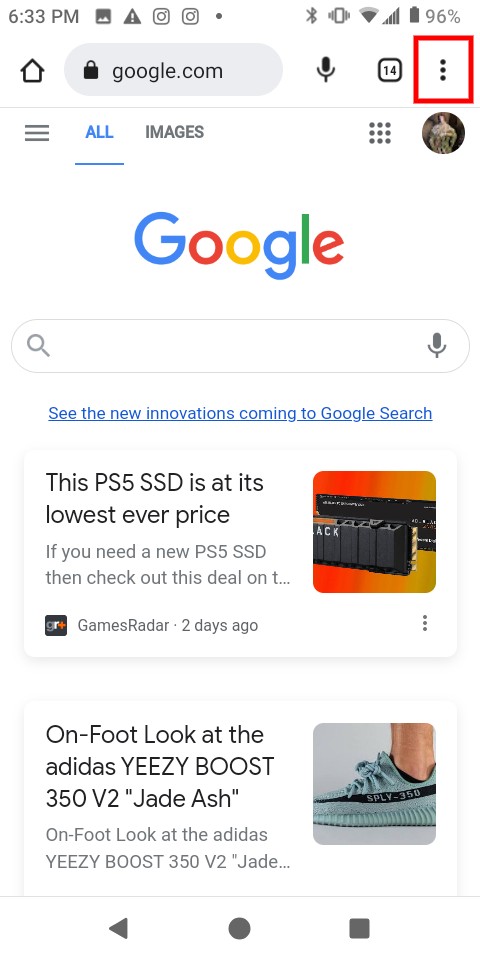The image displayed on a smartphone screen shows a Google search page open in a browser. The phone has a battery life of 96%, indicated by full bars, and the connection signal is at 100%. The time displayed is 6:33 p.m. 

At the top right of the browser, there is a red box outlining the three vertical dots menu icon. Below that, there is a small profile picture of a person. Additionally, the navigation tabs show "All" underlined in blue and "Images" in gray. 

Central to the screen is the prominent Google logo, featuring its characteristic colors: blue, red, yellow, and green. Underneath the logo is the search bar, which includes a magnifying glass icon on the left and a microphone icon on the right. Beneath the search bar, a blue underlined prompt reads: "See the new innovations coming to Google Search."

There are two main advertisements featured. The first ad showcases an image of a PS5 console and the text: "This PS5 SSD is at its lowest ever price. If you need a new PS5 SSD, then check out this deal on the...". This ad is from GamesRadar, posted two days ago. The second ad is for a sneaker, showing an image of the Adidas Yeezy Boost 350 V2 Jade Ash, with the text: "On foot look at the Adidas Yeezy Boost 350 V2 Jade Ash."